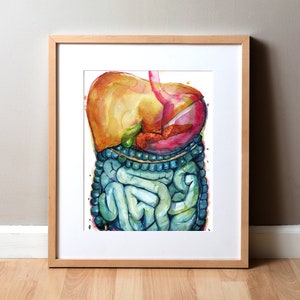The image showcases a framed illustration propped against a taupe-colored wall with light wood flooring. The frame, matching the flooring, is light wood with a white mat. Inside is an eclectic, watercolor-style depiction of the human gastrointestinal system, featuring vivid hues of orange, red, pink, and transitioning into blue and green. The artwork prominently displays the stomach and intestines, artistically rendered rather than clinically accurate, making it appear more as an original, artistic piece rather than a traditional medical illustration.